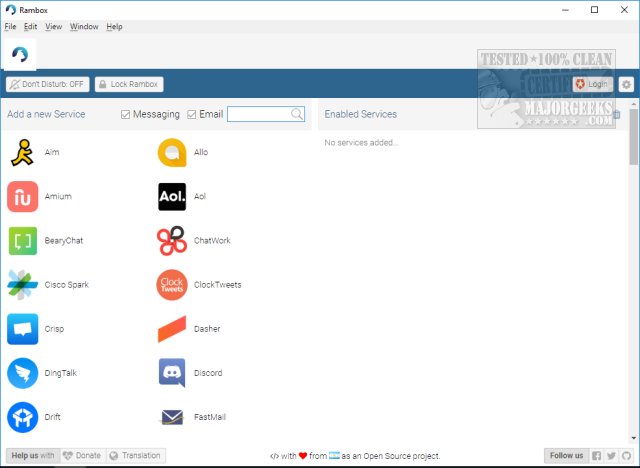The image from the website RamBox features a comprehensive interface with various buttons and icons. At the top, there are menu options for "File," "Edit," "View," "Window," and "Help." A "Do Not Disturb" switch is visible and currently turned off. Adjacent to it is a lock button labeled "Lock RamBox."

Below these settings, there are options to "Add a New Service," categorized under "Messaging" and "Email," both of which are checked. 

On the screen, an array of logos and services is displayed. These include:
- A small, simplistic icon of a stick figure person, drawn in yellow and black.
- The AOL logo, depicted in black and white within a square.
- The ChatWork logo, characterized by a floral design.
- The Clock Tweets logo, featuring an orange circular design with white letters spelling "Clock Tweets."
- The Discord logo.
- The DingTalk logo in blue and white.
- The Cisco Spark logo.

Each of these elements is neatly arranged, providing a clear view of the multiple services integrated into the RamBox interface.